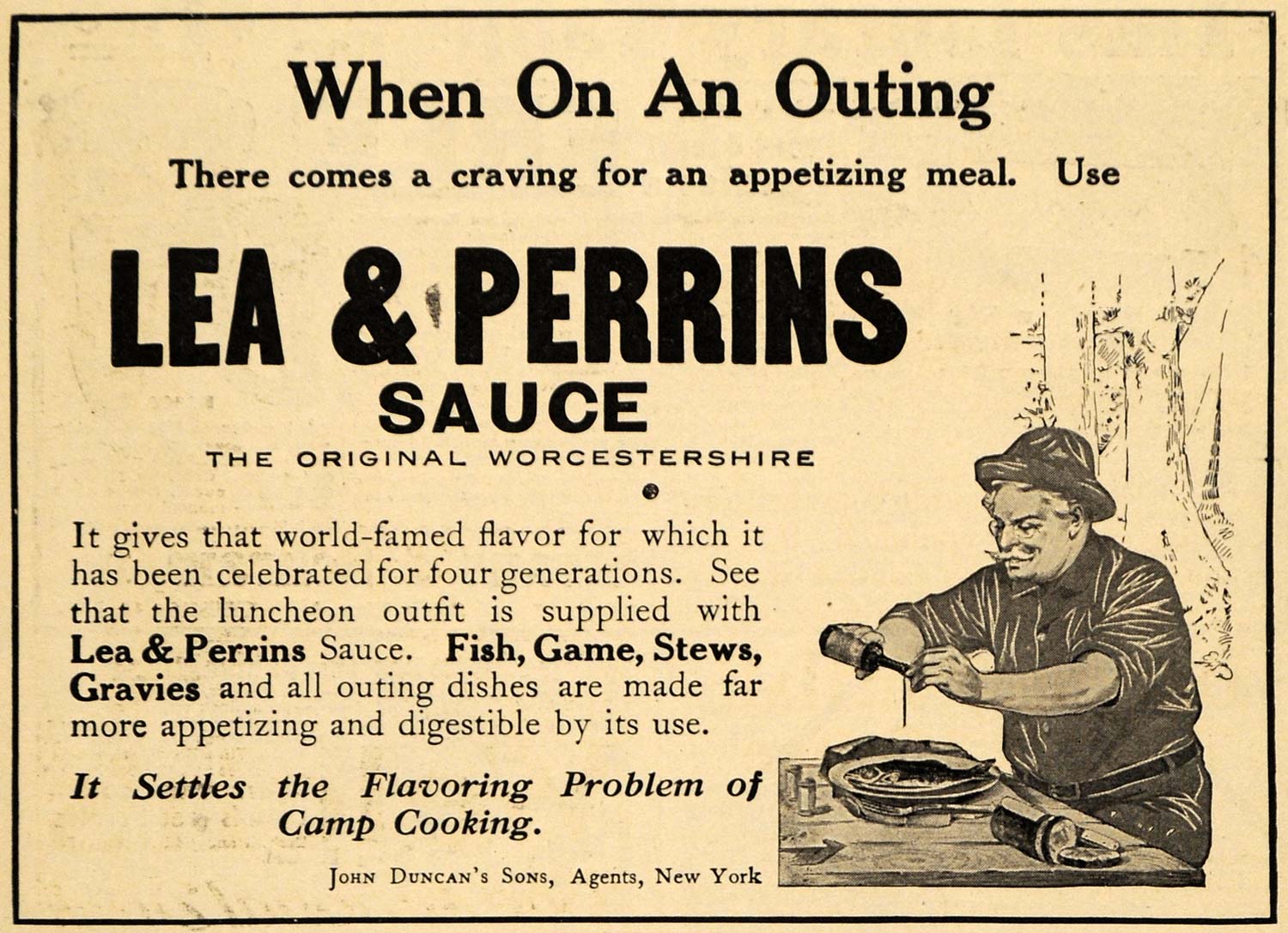This image showcases a vintage sign printed on light brown paper with a bold black outline. The sign features text in black, promoting Lee and Perrin's sauce, famously known as the original Worcestershire sauce. The message conveys that when one is on an outing and craving a flavorful meal, Lee and Perrin's sauce is the perfect choice. It guarantees that world-renowned flavor celebrated for four generations, and it is essential to include in any luncheon outfit. Whether for fish, game, stews, gravies, or any outdoor dish, this sauce dramatically enhances the taste and digestibility, resolving the flavoring challenges of camp cooking. The advertisement is endorsed by John Duncan's Sons, agents in New York. The sign also depicts an older man standing outdoors, likely at a campsite, pouring Lee and Perrin's sauce over a fish, exemplifying its use in an authentic outdoor cooking scenario.